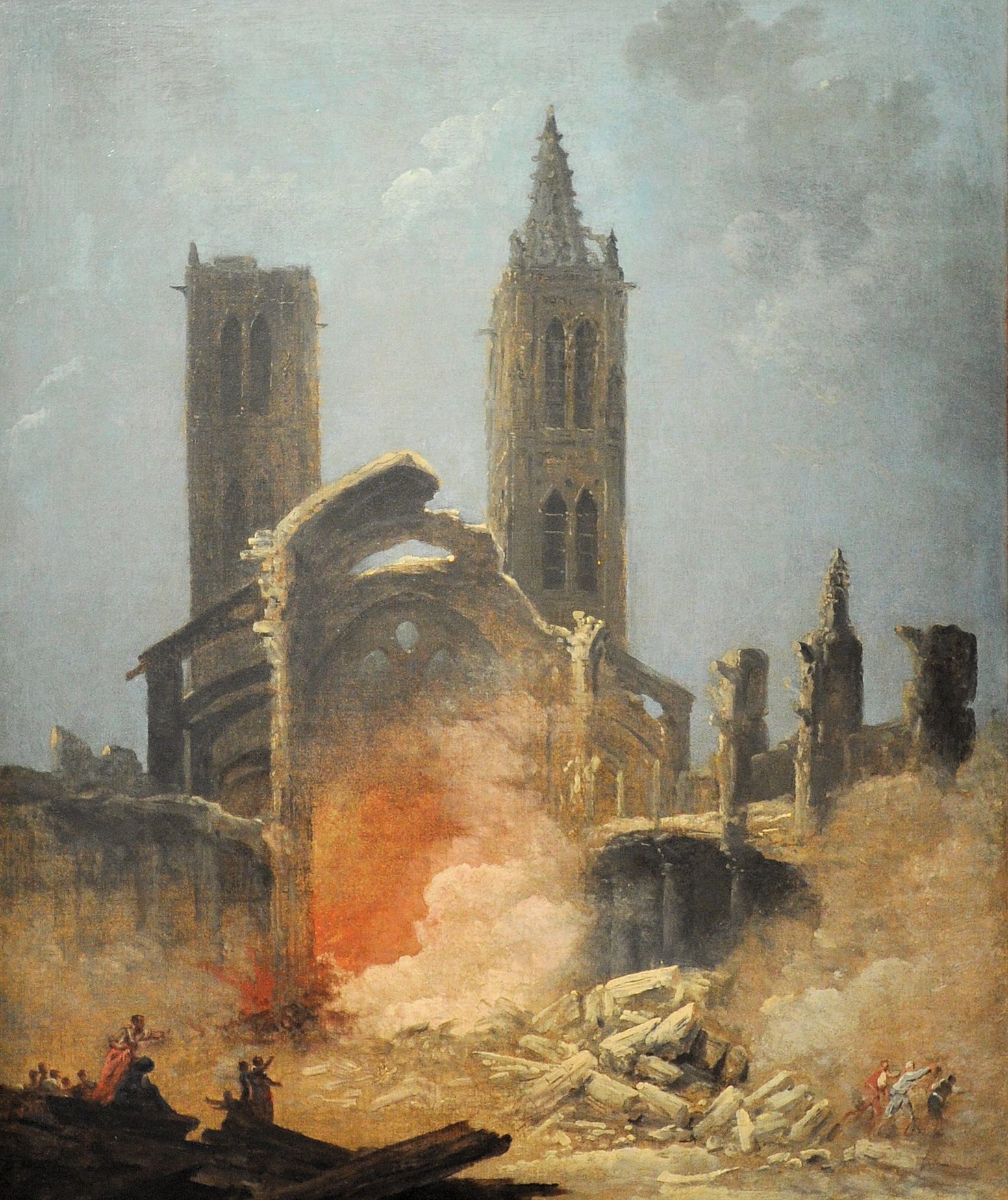In this detailed and somber painting, one is drawn to the scene of a dramatic medieval conflagration, evocative of the historic burning of Notre Dame Cathedral. Dominating the background are two imposing towers, clad in shades of beige and dark charcoal gray. One tower appears intact with its pointy top, reminiscent of the iconic spires, while the other has been partially demolished, its crown conspicuously missing. These architectural giants stand amidst the ruins of a once-grand church, now beleaguered by cascading flames and billowing smoke.

Further in the center, the remnants of the church’s structure are evident, outlined by stark walls from which a destructive fire emanates. The vivid orange hues of the blaze contrast sharply with the otherwise monochromatic background. The immediate foreground is strewn with debris—shattered wood and crumbled rocks—a testament to the recent devastation. Amidst this chaos, a group of eight to ten figures, diminutive yet distinct, gather on rocky outcrops and on the ground. Each figure, robed in garments reminiscent of the Christian era, is engaged in various actions—pointing, watching, and running—away from the fiery ruins.

The painting’s atmosphere is enhancively grim, with a gray, dark sky looming ominously above, interspersed with the occasional glow from the fire's intensity. Surrounding the ruins is a bleak, beige field contrasted by the harshness of the wooden remnants and the sinister red clouds rising from the ground, vividly illustrating the devastation. The visual chaos captures the urgent movement and fear of those witnessing the destruction, many of whom seem to be fleeing the catastrophe. This artful depiction leaves an indelible impression of historical tragedy and human resilience amidst ruin.